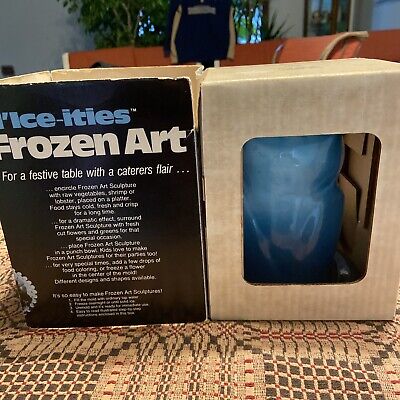The photograph features a packaged item displayed on a cream-colored tablecloth with gray squares and red lines. The focal point of the image is a cardboard box on the right side, which has a transparent window revealing a shiny, blue container or cup inside. The left side of the image displays text in blue and white lettering that reads "Ice Itis Frozen Art," followed by the phrase "for a festive table with a caterer's flair." Additional descriptive text about the product is also visible below the main heading. In the background, the upper portion of several pink chairs is seen, accompanied by some plant life. Completing the scene, a glass door is located in the upper right corner of the image.